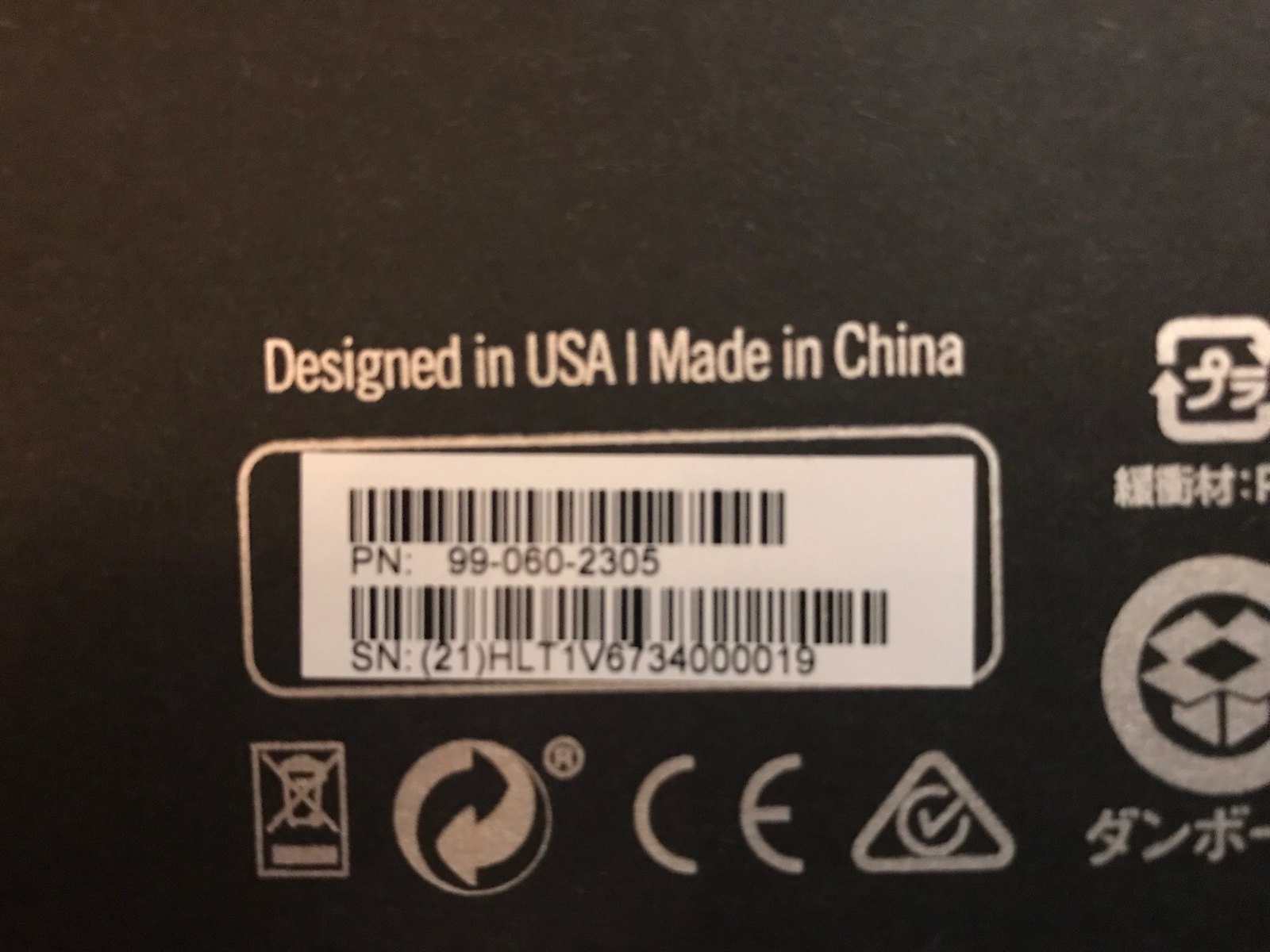This close-up image captures the underside of an electronic device, showcasing its sleek, black surface. Prominently displayed is a barcode on a white label, beneath which the text "PN: [number]" and "SN: [combination of numbers and letters]" is printed. Above the barcode, the label reads "Designed in USA – Made in China" in white ink. A series of unidentified symbols and Chinese characters are also visible, adding to the informational content on the device. Among these symbols, there is a rectangular icon with an item depicted inside it, crossed out to indicate a prohibition, though the specific action prohibited is unclear.